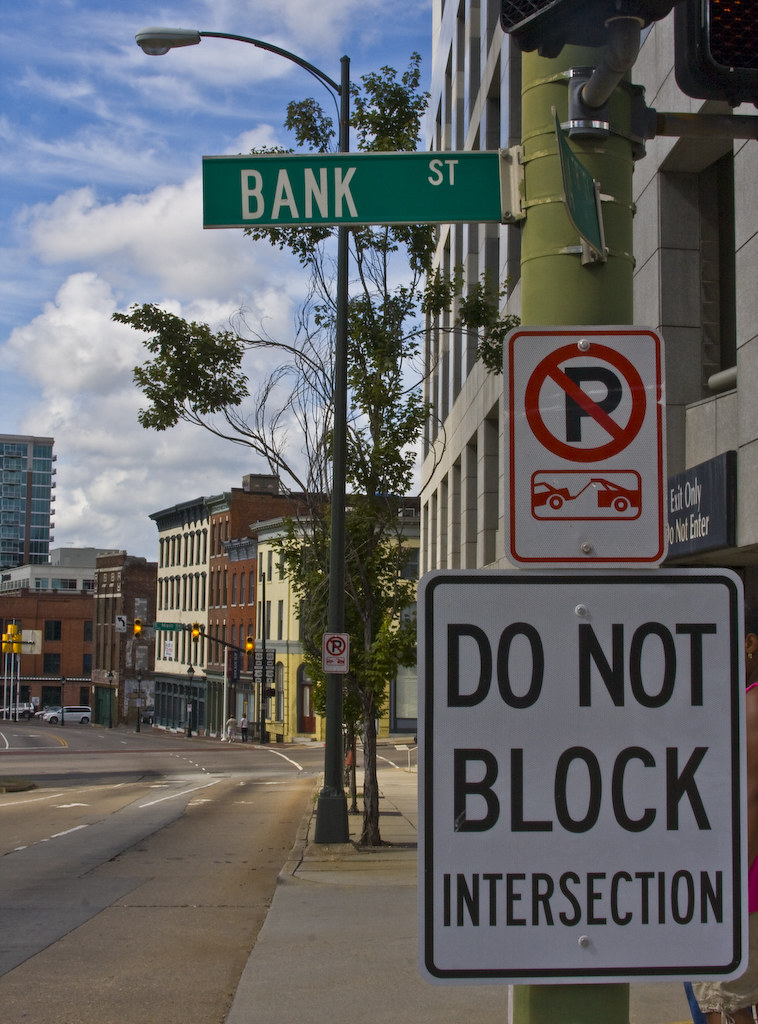This photograph captures a sidewalk scene focused on a green, cylindrical pole adorned with multiple signs. The pole prominently displays a green street sign reading "Bent Street." Directly underneath, a white "No Parking" sign features a black 'P' struck through with a red circle and line, accompanied by a red tow-away vehicle graphic. Further down the pole, another white sign instructs, "Do Not Block Intersection" in bold black letters. To the left of the signs, a street extends into the distance, lined with buildings that create an urban backdrop. The sky overhead is a vibrant blue, dotted with fluffy white clouds, and the scene is punctuated by a couple of trees and a street lamp in the background, adding a touch of natural contrast to the cityscape.